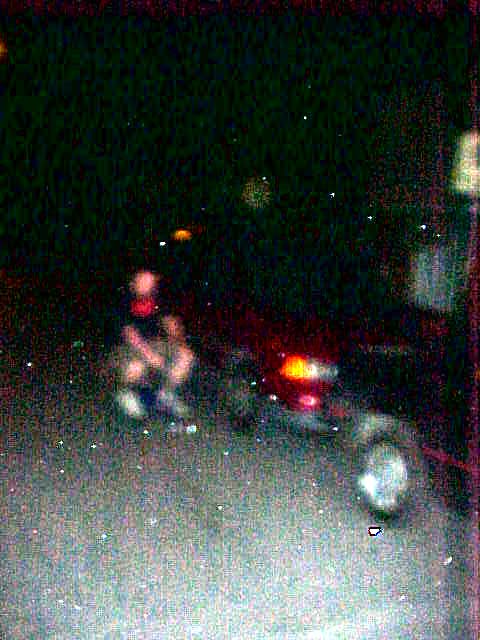In this extremely blurry nighttime outdoor image, we see two cars parked on a pavement beneath a black sky. The car in the foreground is a red sedan with its headlights on, casting a bright orange-yellow and white reflection on the ground. Parked in front of it is a black vehicle, likely a truck, with dark rims featuring silver details. To the left of the red car, a person is crouching in a seated pose. The person has visible shins and white skin, and they are dressed in a black t-shirt with red accents, brownish shorts, white socks, and white sneakers. The ground shows some patchy, snowy green spots. Despite the image's significant blur, reminiscent of low-quality VHS footage, these key details are discernible.